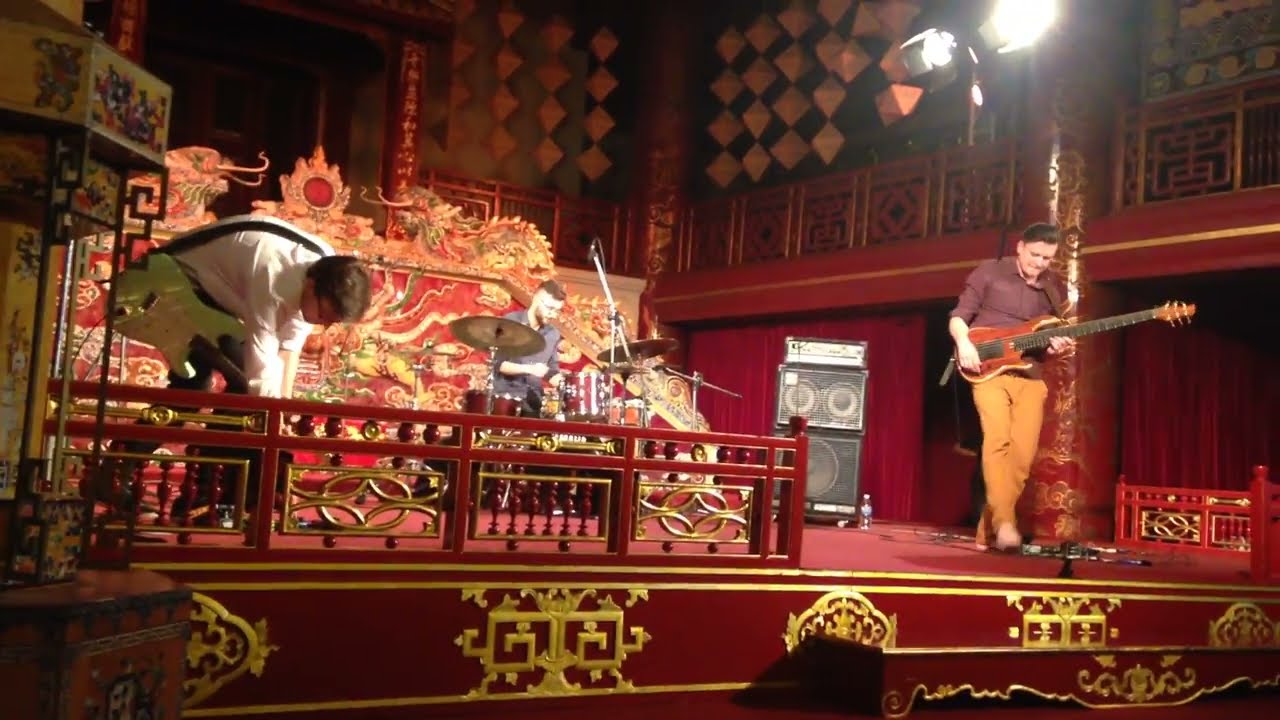The photograph captures an indoor performance by a three-piece band on an ornately decorated stage with a distinct Asian influence, featuring red and gold colors and intricate dragon emblems. The stage, adorned with a red and gold patterned barrier, showcases the band in action. At the center, the drummer, sporting a blue shirt, short brown hair, glasses, and a brown beard, plays a drum set that includes a drum featuring an American flag design. To his side is a bass amp with two small speakers on top and one larger speaker at the bottom.

On the left side of the image, the guitar player is captured mid-adjustment of an effects pedal, holding a green electric guitar with a white pickguard. He wears a white long-sleeve business shirt, black trousers, glasses, and has dark brown hair.

On the right, the bass player, dressed in a brown long-sleeve shirt and mustard-colored pants, stands at the forefront. He plays a six-string bass while looking down at a pedal board. The setting is an indoor music auditorium, bathed in hues of dark red, gold, blue, and other colors, with a light positioned towards the top right corner, illuminating the scene.